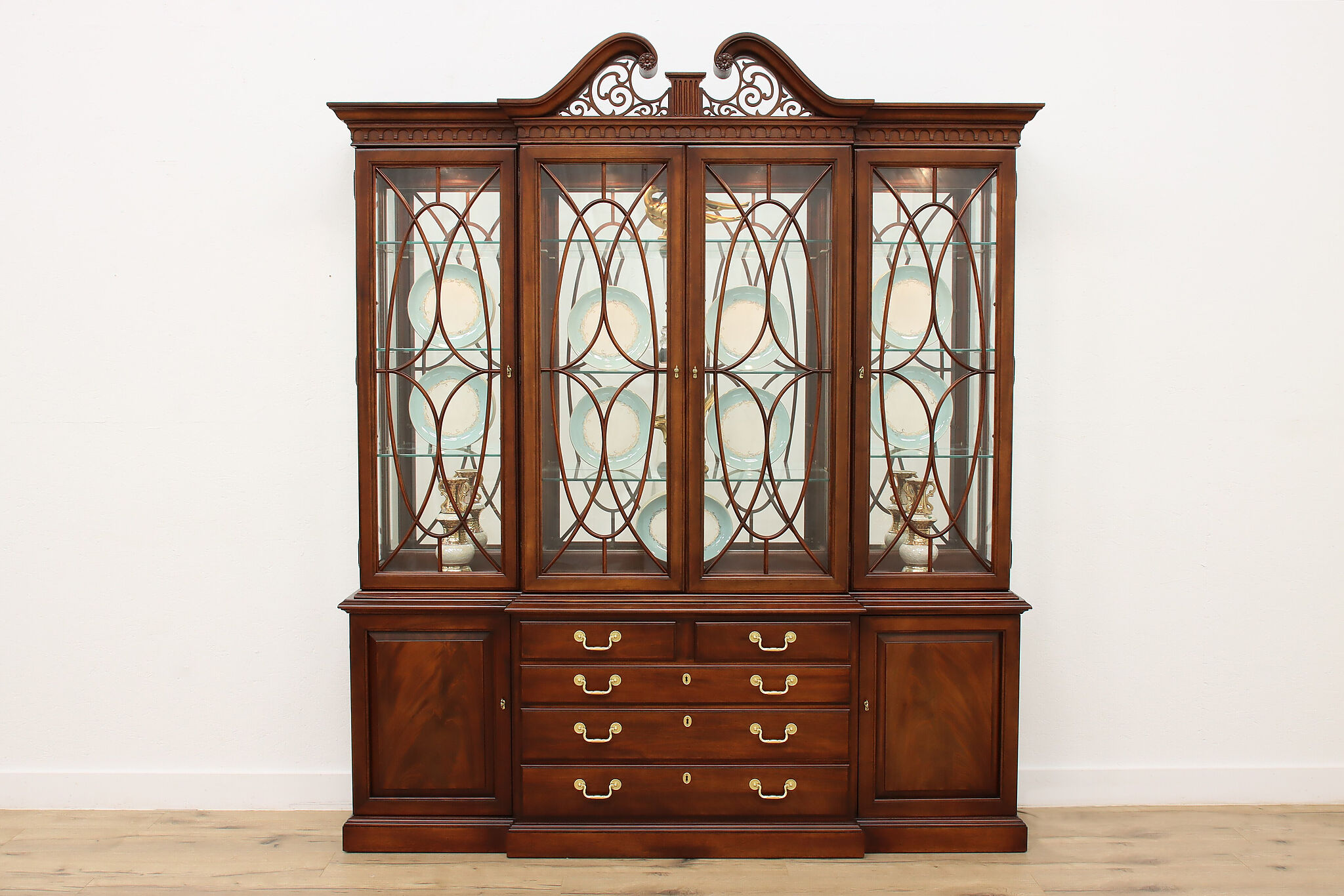The image features a classic, dark brown wooden and glass china hutch reminiscent of a traditional piece you might find in a grandmother's home. The hutch stands against a plain white wall on a light brown floor. At the bottom, the hutch includes two wooden doors on either side, framing a central column of four drawers. The top row of drawers is split into two individual compartments, while the lower three are single drawers, each equipped with gold handles and lockable for secure storage.

The upper section of the hutch is characterized by glass doors encasing three glass shelves. The glass doors have a distinctive wooden framework forming an oval, egg-like pattern when viewed from a distance, enhancing its ornate appearance. Inside, the glass shelves are adorned with a single white dish on each of the three shelves and additional dishes appear on each rack, totaling four visible plates per rack. Reflecting at the back is a mirror, amplifying the elegance of the displayed china. The top of the hutch is also embellished with a spiral-like wooden design, adding a decorative flourish to this timeless furniture piece.